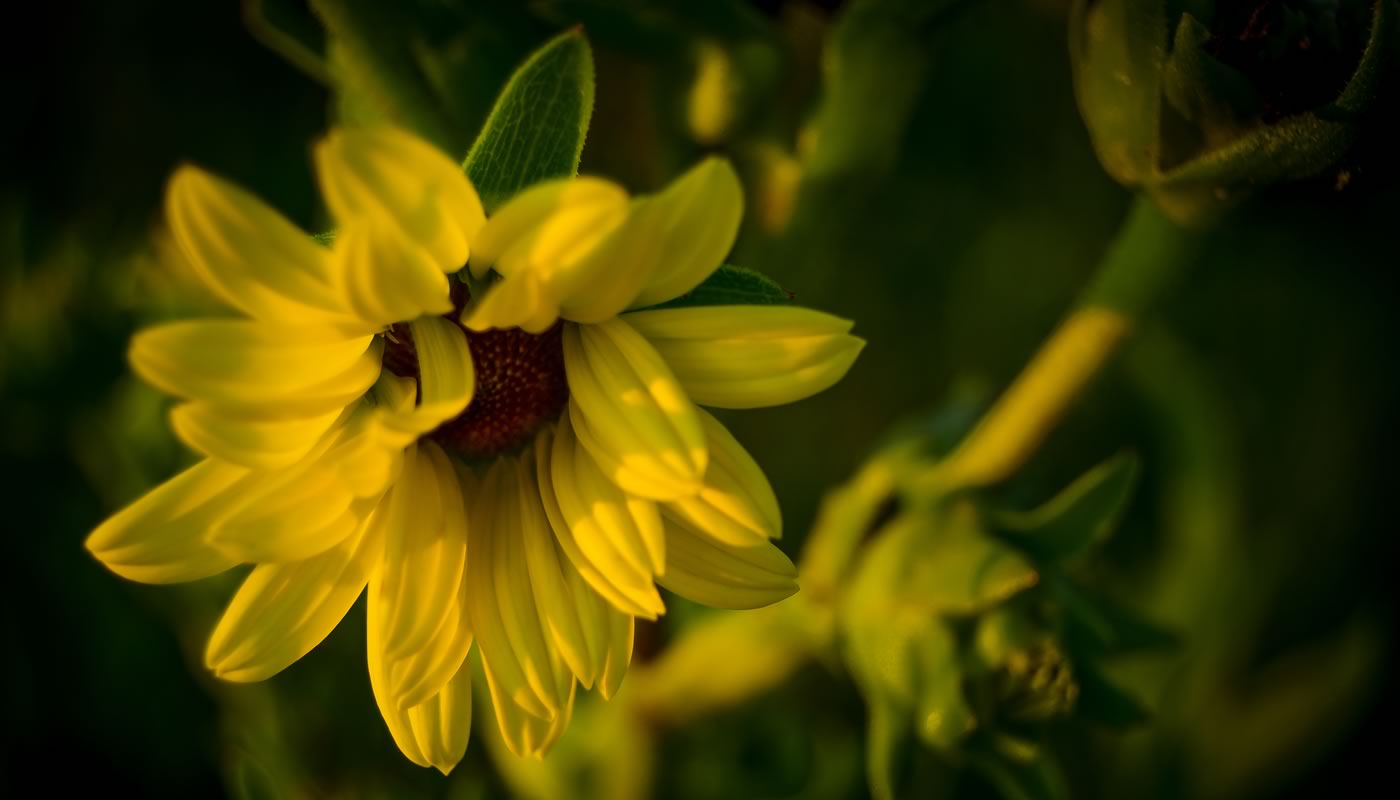The image is a stylized depiction of a lovely daisy set against a dark background, which accentuates the delicate details of the flower and various foliage. The daisy, which is positioned prominently in the forefront, is around three-fourths open. Its petals, which are yellow and pointed, branch out in all directions but still partially enclose its bright orange, grainy center. The petals appear almost translucent near the tips and have multiple small ridges. Some green flower leaves stick out above the daisy, and there are blurred stems to the right, suggesting another daisy that has yet to bloom. The scene, evoking a sense of spring, features sunlight that is not very bright, indicating it might be morning or evening. The background is mostly dark, with hints of other out-of-focus flowers and plants, adding depth to the composition.